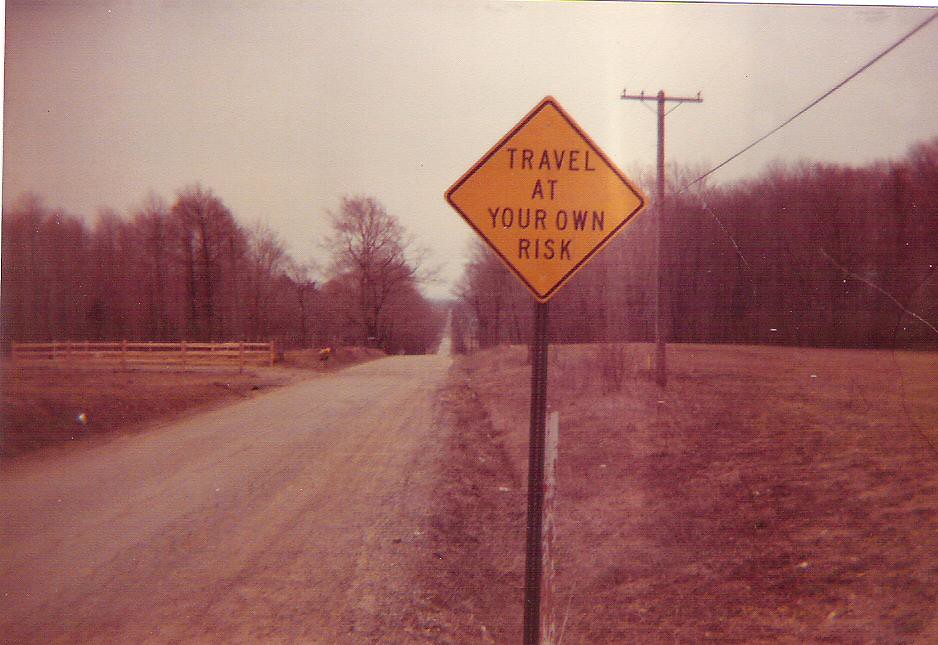In this sepia-toned photograph of a rural landscape, a vivid yellow diamond-shaped traffic sign stands out near the roadside, warning "Travel at Your Own Risk." The unmarked, hilly country road meanders through fields that stretch on either side, eventually leading to a densely forested area in the distance. On the left side, a sturdy brown slatted fence encloses part of the field, while telephone poles on the right side of the road connect with overhead wires that follow the road's undulating path.